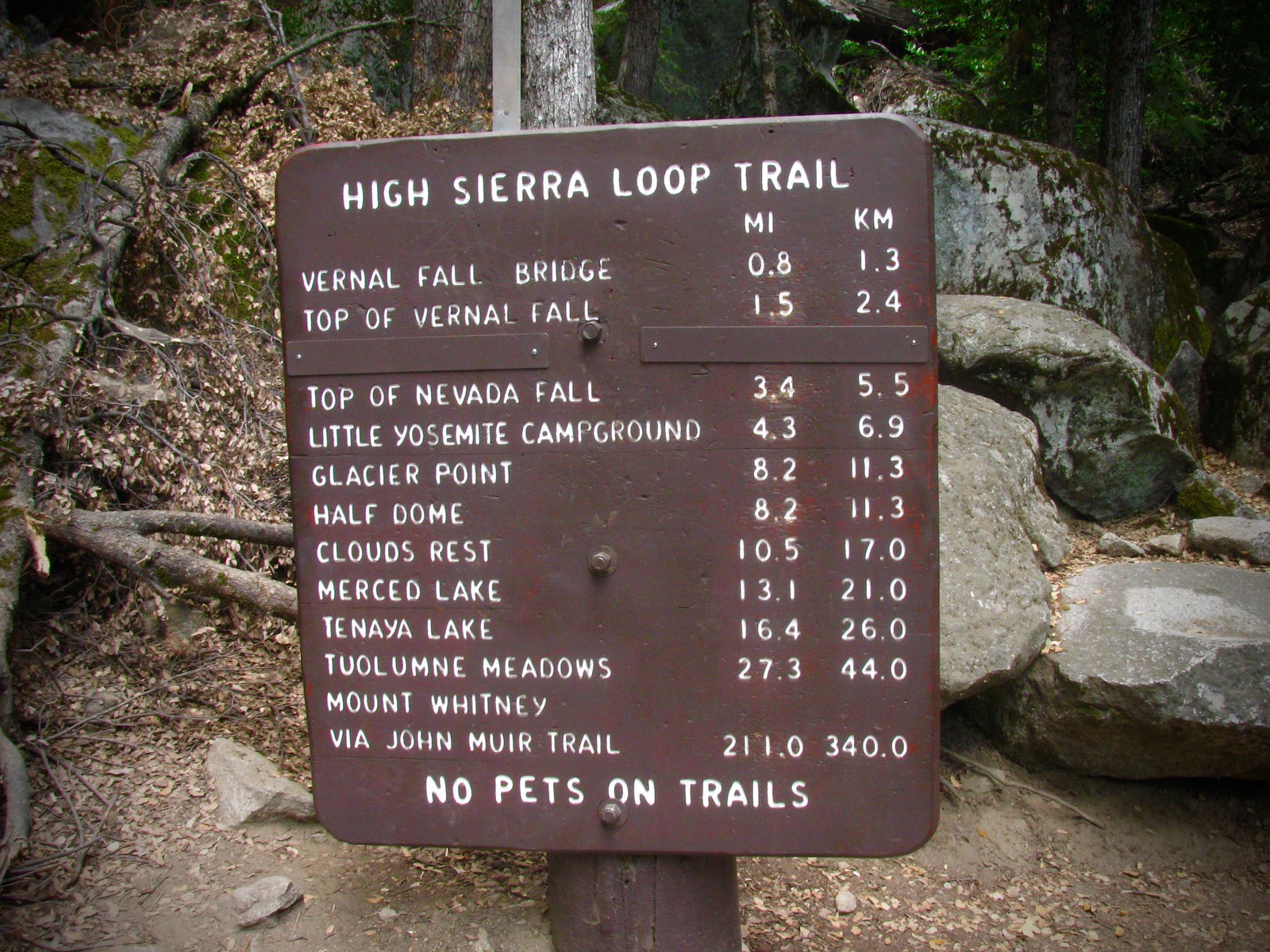The photograph captures an outdoor scene of the High Sierra Loop Trail sign, firmly mounted on a wooden post amidst natural surroundings. The background is a picturesque combination of large and small rocks, standing trees with vibrant green leaves, and fallen trees covered in old leaves. The brown metallic sign, bolted at the center, stands prominently in the foreground. The sign features white lettering that lists various landmarks and their respective distances in both miles and kilometers: Vernal Fall Bridge (0.8 miles, 1.3 km), Top of Vernal Fall (1.5 miles, 2.4 km), Top of Nevada Falls (3.4 miles, 5.5 km), Little Yosemite Campground (4.3 miles, 6.9 km), Glacier Point (8.2 miles, 11.3 km), Half Dome (8.2 miles, 11.3 km), Clouds Rest (10.5 miles, 17 km), Merced Lake (13.1 miles, 21 km), Tenaya Lake (16.4 miles, 26 km), Tuolumne Meadows (27.3 miles, 44 km), and Mount Whitney via John Muir Trail (211 miles, 340 km). The sign prohibits pets on the trail with a message at the bottom. The natural backdrop of the trail adds a serene and scenic context to the informative signpost.